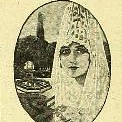This is a small, vintage photograph set in an oval frame, featuring a woman wearing an elaborate white headdress that drapes down below her chin, reminiscent of a veil or crown. Her face is clearly visible, and she gazes directly at the viewer with small lips and dark eyes. Behind her, a fountain can be seen, along with trees and a tower emerging from the foliage in the distance. The image, though appearing yellowed with age rather than strictly black and white, has an ivory-colored background that enhances its antique feel. The photograph is blurry, adding to its aged and mysterious aura.